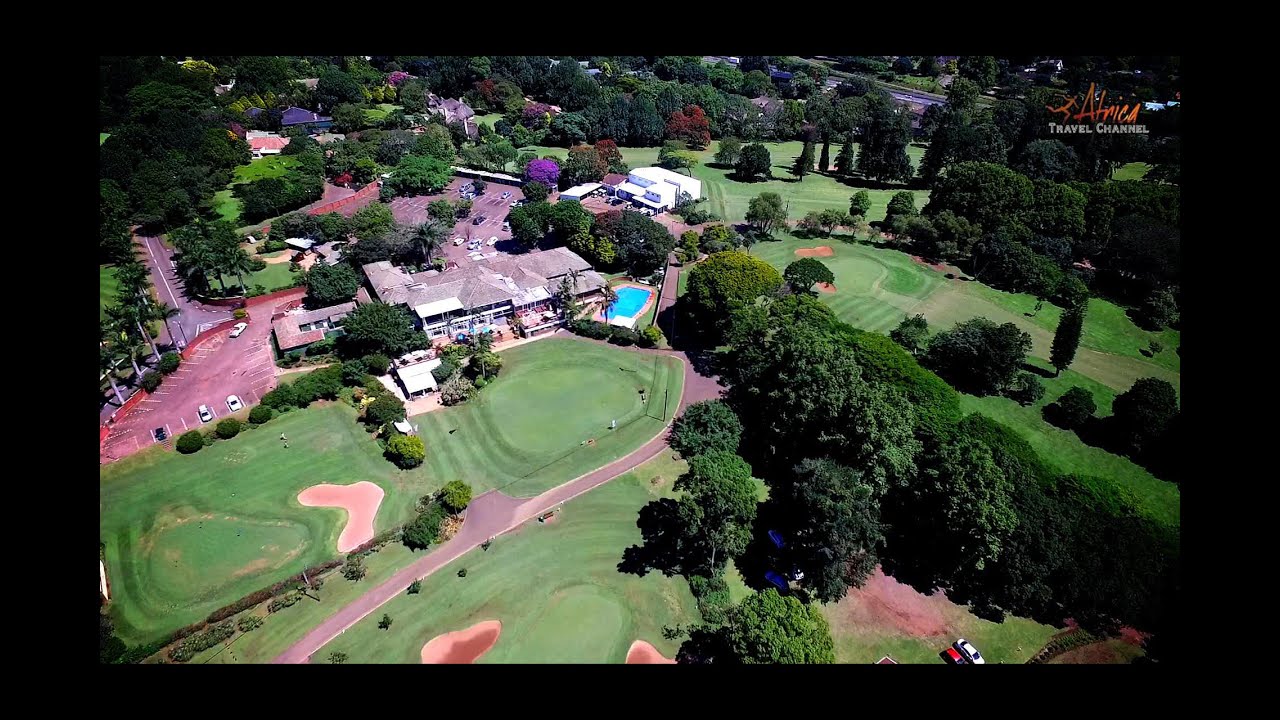The image appears to be an aerial view, possibly a still frame from a video, taken from a high vantage point, such as a drone or helicopter, capturing the expansive landscape of a country club or golf course. The focal point is the lush green golf course, which dominates the foreground and middle areas of the picture, particularly on the left side. The course features distinct lighter and darker green grass, indicating different cuts, along with several clearly visible sand traps. Toward the upper left and middle of the image above the greens, there is a brown-roofed clubhouse, a large building nearly centered in the frame, surrounded by a parking lot and a pool to its right. Extending beyond the main facilities, more buildings are interspersed among dense clusters of green trees. Residential areas and various infrastructure elements like roads and driveways can be seen in the distant background. The colors in the image range from vivid greens and browns to blues, grays, and off-whites, suggesting a vibrant daytime setting. Additionally, the top right corner of the frame includes the visible text "Africa Travel Channel," indicating a possible broadcast origin. A black border surrounds the top, sides, and bottom of the image, hinting that this could be a photograph of a TV screen.